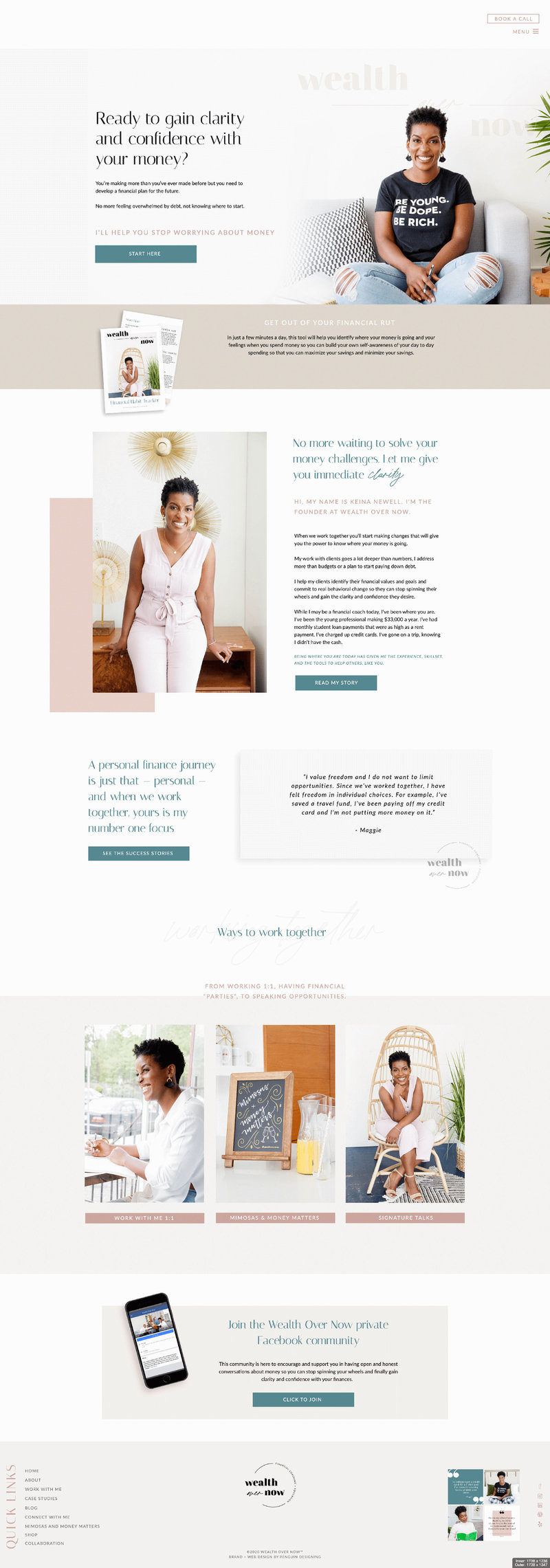Here is a cleaned-up and detailed caption for the image:

---

This screenshot captures a section of a website designed to offer financial planning services. The top of the page features a light gray background. To the right, there is a button with a light brown border labeled "Book a Call," and next to it a menu icon represented by three horizontal lines stacked vertically.

Moving down, the background transitions to a slightly darker shade of gray, still light in tone. Centered on this background is the word "Wealth." Flanking this, on the left side in dark brown text, is a compelling headline: "Ready to gain clarity and confidence with your money?" Below this, additional text reads, "You’re making more than you’ve ever made before, but you need to develop a financial plan for the future. No more feeling overwhelmed by doubt, not knowing where to start." 

At the page's bottom section, text in dark brown promises, "I'll help you stop worrying about your money," followed by a teal call-to-action button labeled "Start Here."

On the lower part of the page, there is an image of a woman casually sitting on a couch. She is dressed in a black t-shirt, ripped jeans, and black dangly earrings. Below this, a taupe-colored banner displays two pamphlets stacked together, stating, "Get out of your financial rut."

Further down, another white banner with teal text declares, "No more waiting to solve your money challenges. Let me give you immediate clarity." This is followed by a personal introduction: "Hi, my name is Kiana Newell. I'm the founder at Wealth Over Now," accompanied by a brief professional description.

Continuing, there is another banner emphasizing the personalized nature of the financial guidance provided: "A personal finance journey is just that, personal. When we work together, yours is my number one focus." Centralized text explains, "Ways to Work Together," next to additional images.

The page concludes with an invitation to join a community: "Join the Wealth Over Now private Facebook community."

---